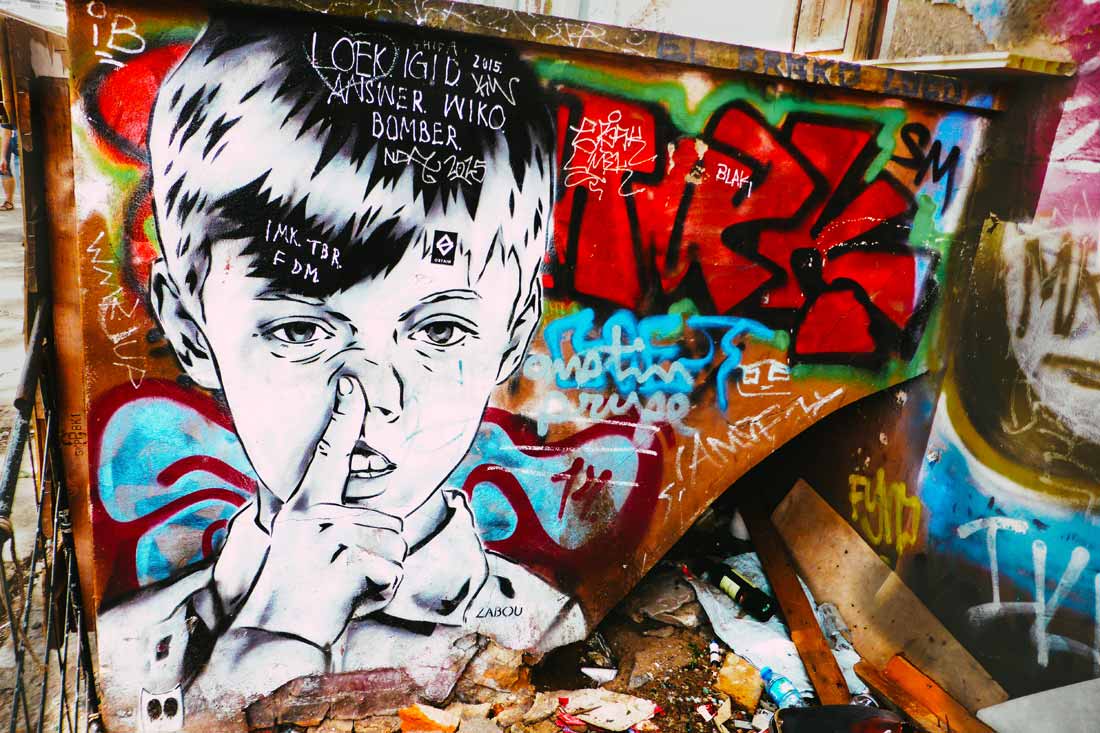The photograph showcases a vibrant and gritty scene, dominated by a graffiti-covered dumpster spanning the entire length of the image. Central to the composition, slightly to the left, is a striking black-and-white rendering of a young boy with a short haircut, depicted picking his nose with his right hand. His lack of color stands in stark contrast to the vivid, multicolored graffiti surrounding him, including red and blue elements. The boy's image features white, non-English text in his hair. Flanking the dumpster are graffitied walls, enhancing the rebellious urban atmosphere. The ground surrounding the dumpster is littered with trash, wood, wine bottles, and food, suggesting an abandoned or neglected location, possibly an alley or under a bridge.